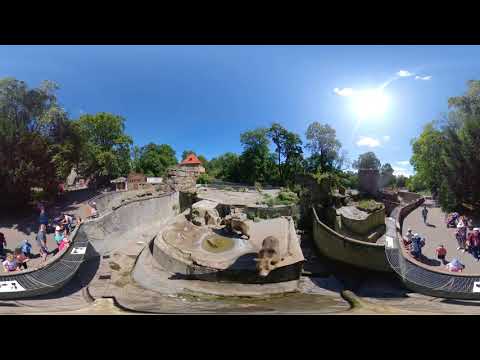This image captures an aerial zoo scene on a bright, sunny day with a clear blue sky and a few scattered white clouds. The photograph is framed by black borders at the top and bottom, occupying about 10% of the frame. Central to the image is a bear enclosure with rocky terrain, including a prominent rock where one brown bear is lounging, while another bear walks away in the background. There's a circular area with water and some green patches, accompanied by various plants.

The enclosure is surrounded by a U-shaped walkway where 20 to 30 people, including adults and children dressed in colorful clothing, are gathered. Some are taking pictures, and others are observing the bears. The walkway is bordered by a barrier, ensuring safety as visitors view the animals. To the right of the walkway, several small, pagoda-like huts can be seen, and an orange-roofed building is visible in the background. The scene is bathed in sunlight, especially prominent on the right side of the image, creating a bright and inviting atmosphere. Lush trees add to the natural ambiance, contributing to the overall depiction of a lively day at the zoo.